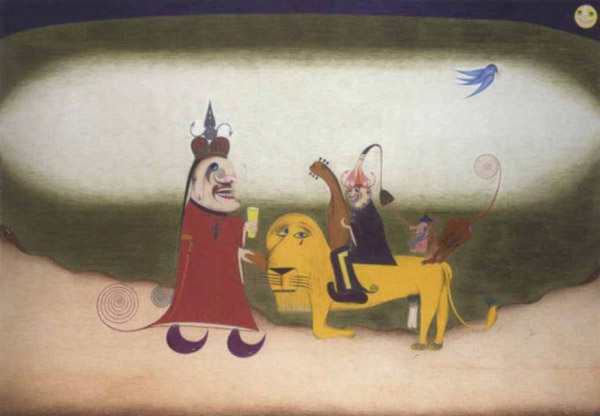In this intricate painting, a peculiar scene unfolds against an abstract background with a light brown oval centerpiece and a dark green-and-brown border, suggestive of a forest. Dominating the scene is a yellow lion with asymmetrical eyes, one of which has a tear. The lion is ridden by a court jester dressed in purplish-black attire, adorned with a pink, tasselled hat. The jester holds a stringed instrument and appears to be serenading.

In front of the lion stands an emperor-like figure, attired in an opulent red robe that spirals extravagantly at the hem. The emperor has a face resembling makeup with a broad mustache, and his curved, crescent moon-shaped shoes add a whimsical touch. A brown crown with silver-tipped arrows adorns his head, while his long black ponytail flows behind him. The emperor's mouth is open, facing the lion, as if in conversation or command.

Behind the lion, a small monkey with a spiraled tail lingers, adding another layer of oddity to the tableau. Above the scene flies an abstract bluebird with elongated wings and tail, and a smiling moon looks down from the sky. The characters appear to be traversing a light brown road within the central oval of the painting, contributing to the scene's surreal and fantastical ambiance.